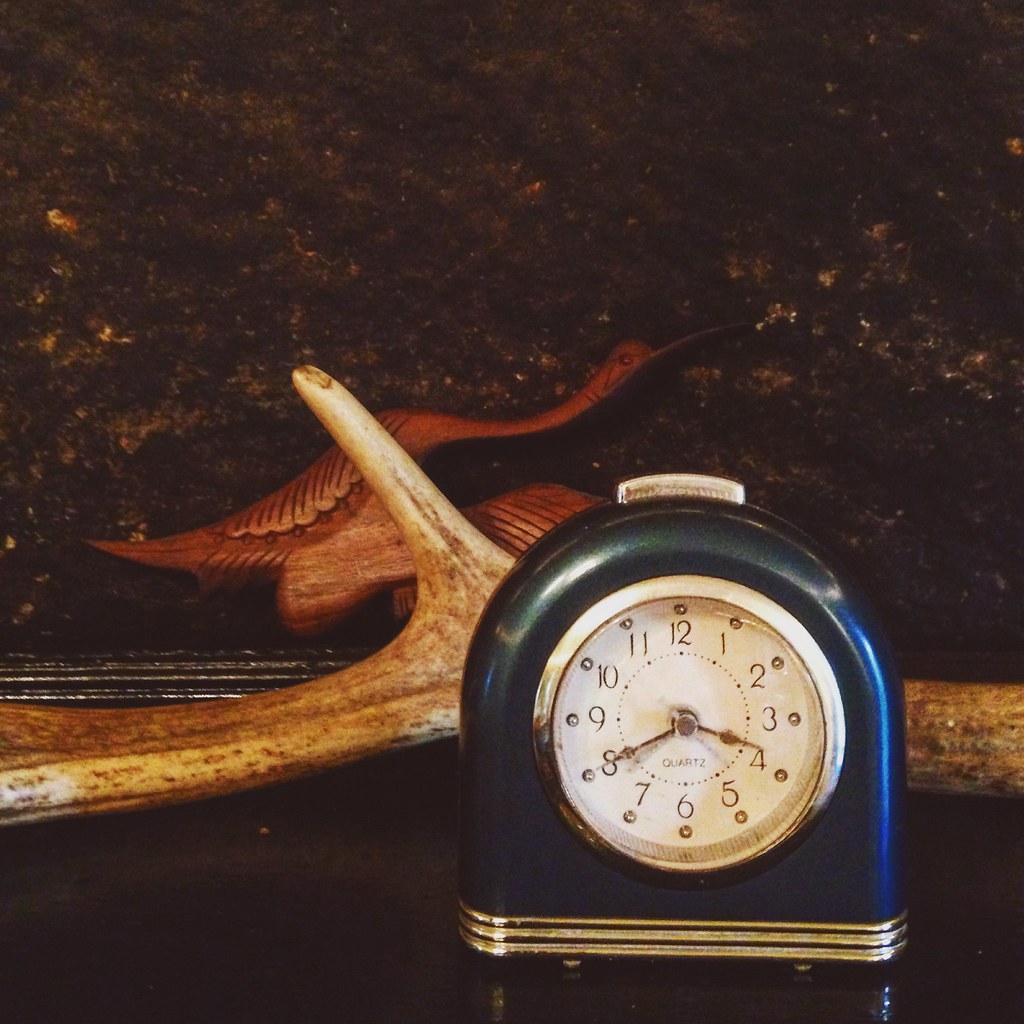The image is a square, vintage-style color photograph, likely taken using film or possibly as a slide. The colors in the image are slightly dulled, with low saturation and low contrast, giving it a flat appearance. At the focal point of the photograph is a blue and green travel alarm clock, distinctly shaped like half an arc with a flat bottom and a curved top. The clock features a large button on its top and has a round face that appears white or yellowed with age. Its time is indicated by black hands and bold black numbers. The clock stands on a mantle, positioned in front of a piece of driftwood. The background features a wall adorned with a mural that includes the image of a wooden bird. This bird is characterized by its long neck and elongated beak.